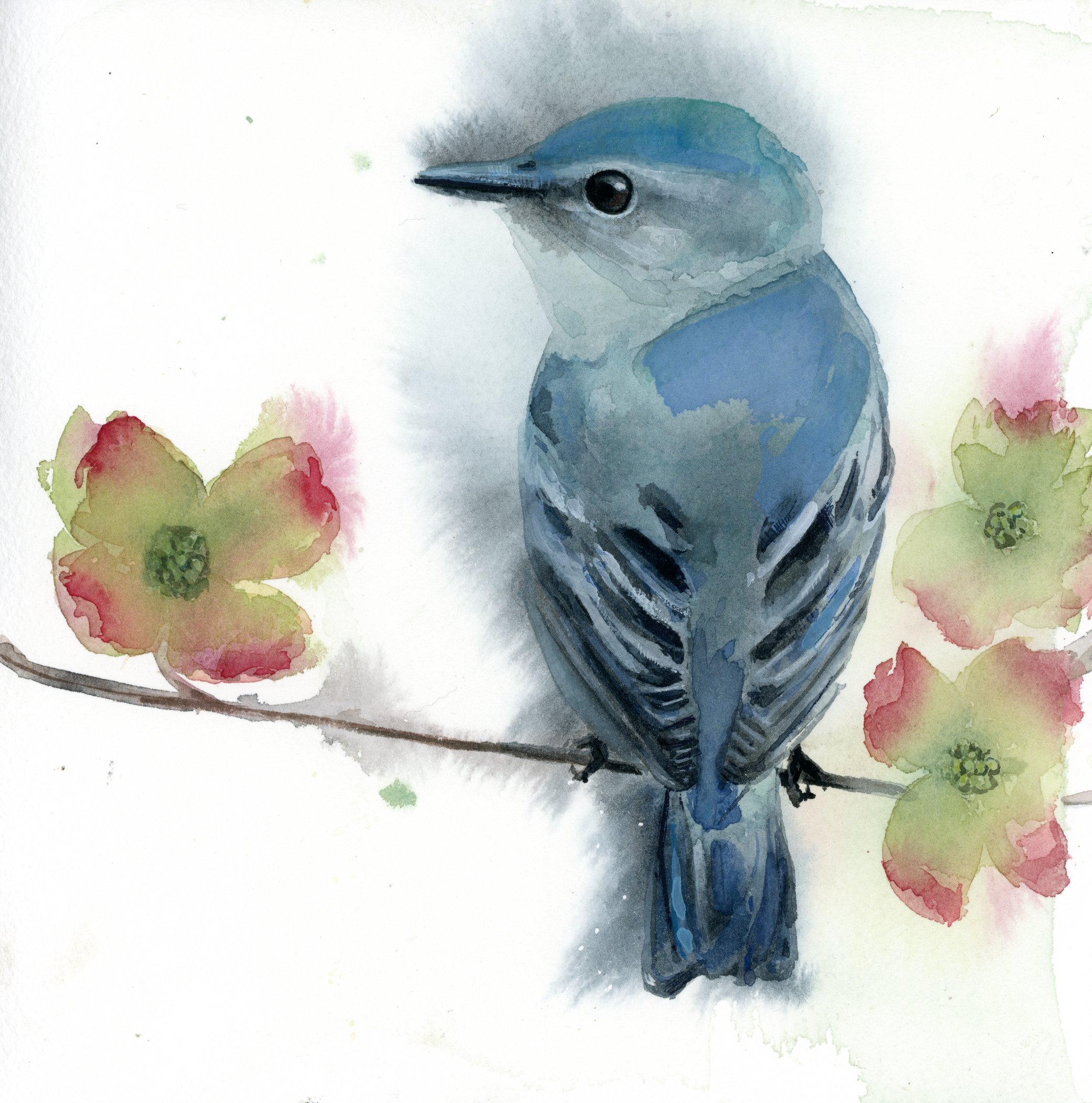This is a detailed watercolor painting of a bluebird, exquisitely standing on a slender branch. The background is completely white, allowing the vibrant colors of the bird and flowers to stand out. The bluebird, which resembles a blue jay, is perched closer to the right side of the image. Its plumage showcases a stunning blend of sky blue and aquamarine tones on its head, body, and tail, with a white neck and distinctive black and white stripes on its back. The bird’s beak and eyes are both black, adding to its lively expression as it faces left, displaying its left eye and giving the composition a dynamic feel.

The thin branch starts just below the mid-height of the image on the left side, extending downwards towards the right. Adorning the branch are delicate flowers that look reminiscent of plum blossoms, each with a green center transitioning to white petals tipped with pink hues. There is one flower to the left of the bird, situated at the end of the branch. To the right of the bird, there are two flowers stacked vertically—one almost in line with the branch and another just above it. The arrangement of the bird and flowers, along with the intricate details and color transitions, creates an enchanting and harmonious scene.